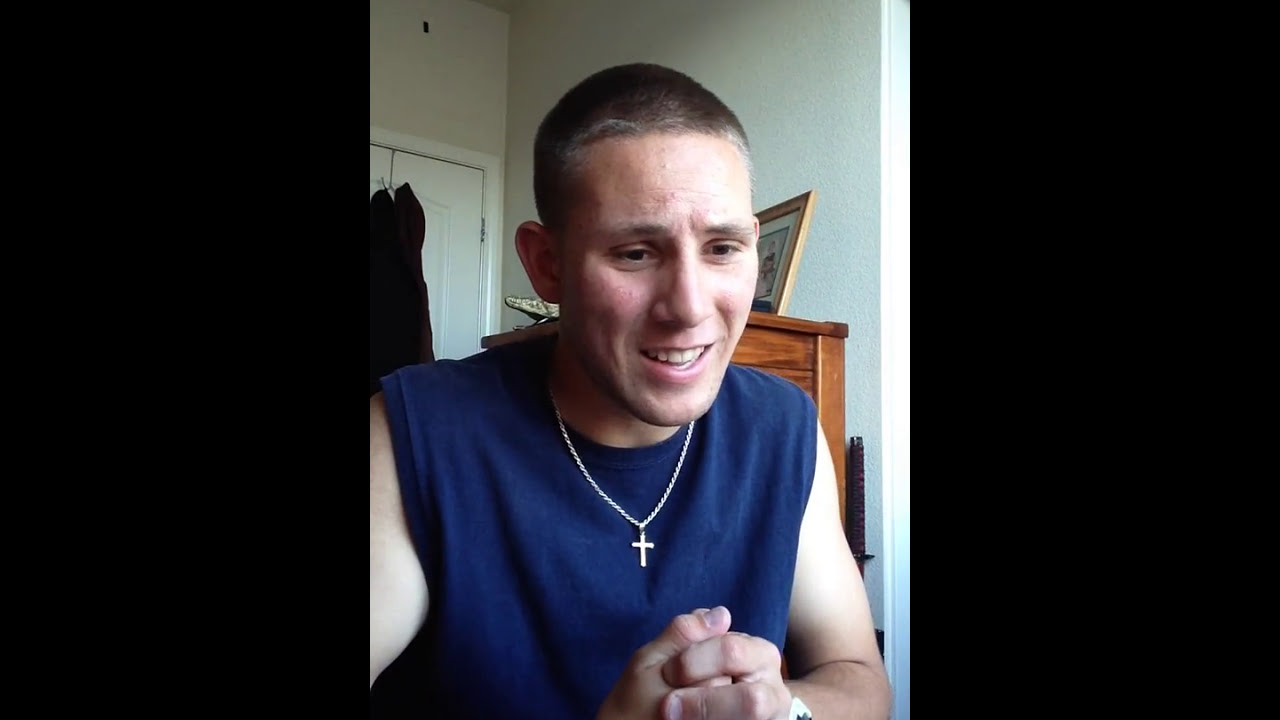The image features a young Caucasian man, likely in his early 20s, situated prominently in the center. He has very short, almost buzz-cut brown hair with slight hints of gray in the front, and brown eyes. His expression appears to be a combination of a slight smile and concern, as if he is engaged in a conversation or video chat. The man is dressed in a blue, sleeveless sweatshirt with a circular collar, and he wears a silver chain necklace with a cross that hangs about halfway down his chest. Additionally, he sports a watch with a white band on his left wrist.

He is positioned against a backdrop of a white wall, with a wooden dresser stained a dark tan color behind him. A picture frame sits atop the dresser, and a closed closet door is to the side, with a black coat or garment hanging on it. The image is framed by two black rectangles on either side, giving the impression of a bordered or split-screen effect. The overall setting appears to be a bedroom.